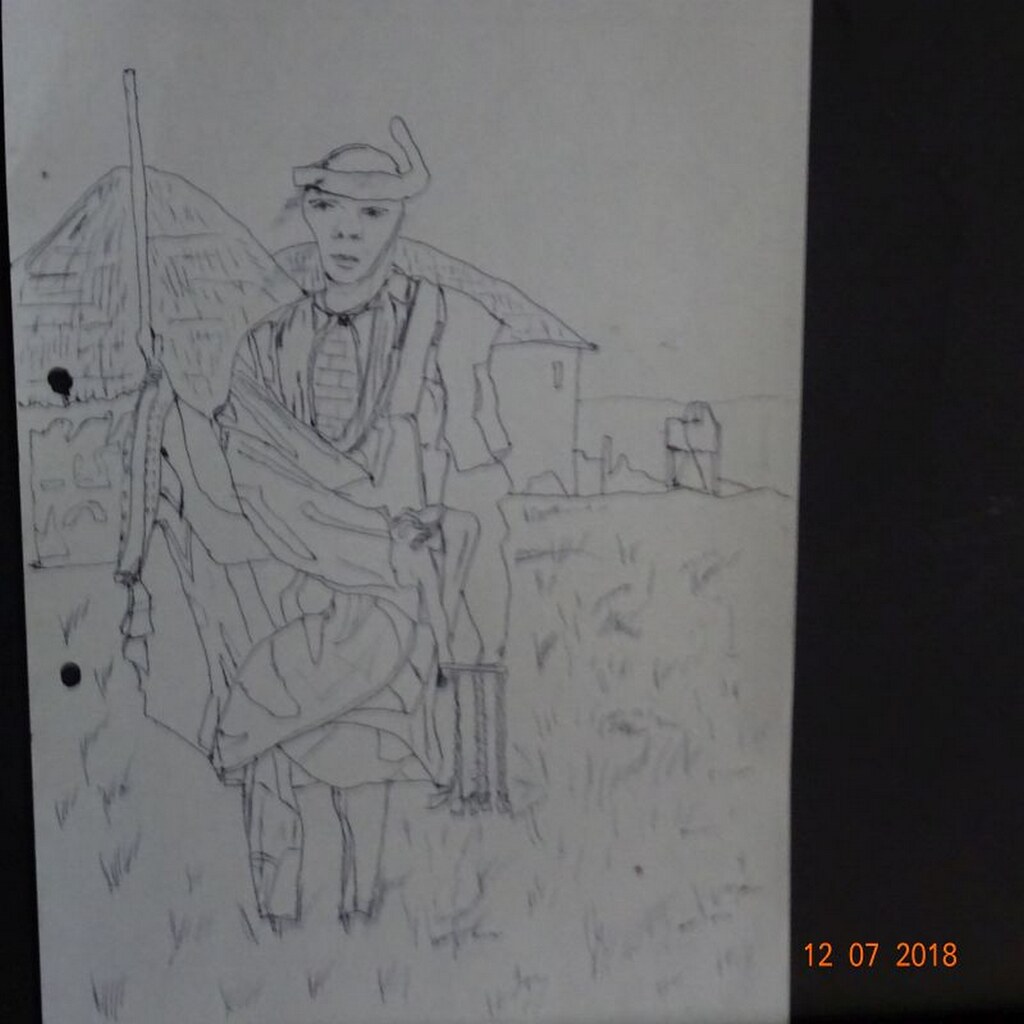The photograph captures a detailed black and white drawing on a two-hole sheet of lined white paper, though the lines are faint and barely visible. The paper rests on a dark, likely black surface, with a date stamp "12-07-2018" in orange at the bottom right corner, indicating the photograph was taken on December 7, 2018. The drawing, made with black ink, features a figure standing in the foreground, possibly an African tribal member or warrior. The figure is heavily dressed in robes or multiple layers of clothing, with a staff in his right hand and additional garments draped over his left forearm. Surrounding the figure is a field, represented by small lines indicating grass. In the background, there are various structures: thatched-roofed, circular buildings resembling traditional huts, a broken wall, part of a house, and a distant tower structure with lines suggesting hills on the horizon. The image is slightly blurry, adding to its hand-drawn aesthetic.